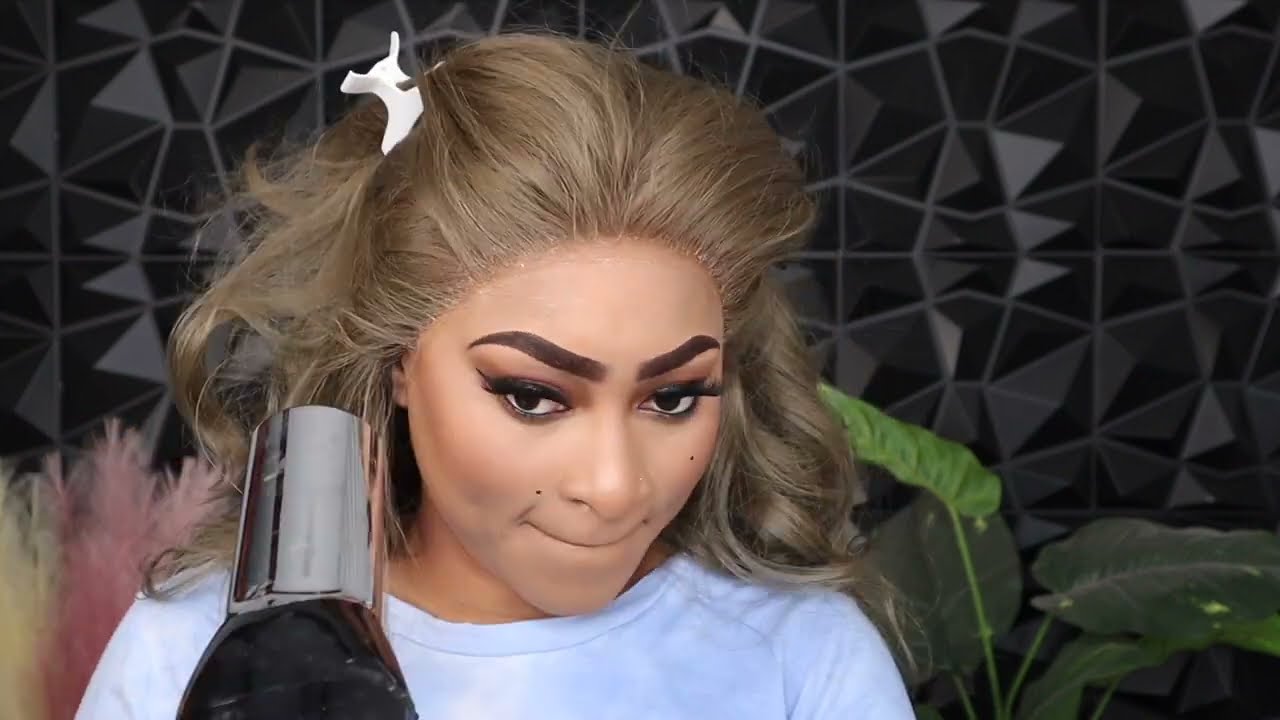The photograph depicts a woman with wavy blonde hair, partially held back by a small white clip, as she uses a black blow dryer with a silver tip on her hair. Her heavily made-up face features dark, thick, painted-on eyebrows and two beauty marks—one above the left side of her mouth and another on her right cheek. Her light blue shirt is visible in the image where only her head and the upper part of her shoulders can be seen. The background is a geometric design of black and gray, including a potted plant with large green leaves on the bottom right, and some pink feathers peeking in from the left side. Additionally, there's a cropped bottle of nail polish with a silver cap on the left side of the image.